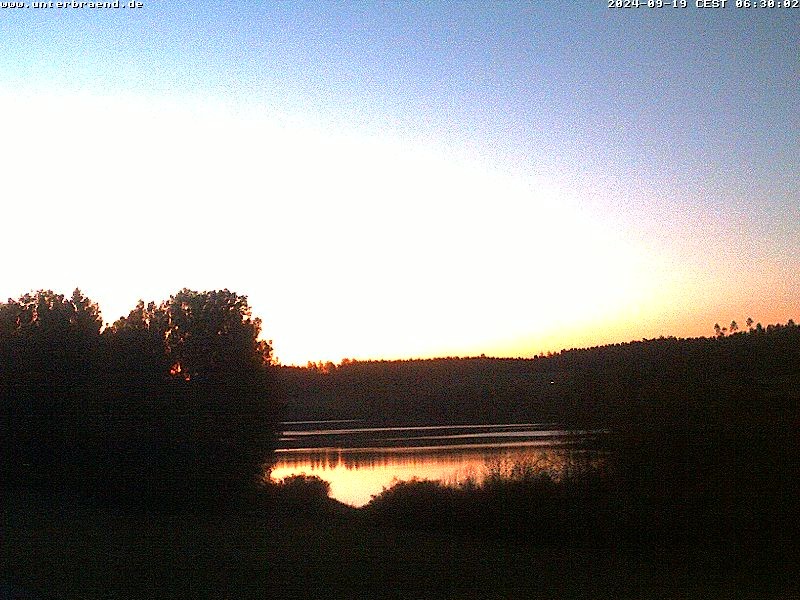The image is a horizontal rectangular photograph capturing a serene countryside scene at sunset. In the immediate foreground, there is a well-manicured grassy area where the photographer stands. A concrete path, yellow-tinted and intersected by large thistles of grass, runs horizontally across this grassy expanse. The path separates the foreground from a downward sloping hillside that leads to a peaceful lake featuring rippling, dark brown water, encircled by possibly stone-covered edges.

To the left of the image, trees with fewer leaves and brownish hues contrast sharply with the more densely packed and green-leaved pine trees visible in the far background. On the right side of the photograph, there is dense brush and darkened foliage, contributing to the overall dimness of that area. The sky dominates the upper part of the image with overcast gray clouds, indicating the sun has already set in another direction, yet casting a lingering daylight over the scene.

The image is timestamped in the top right corner with the date "2024-04-07 CEST" and the time "16:45:02." In the same corner, the text "www.unterbrenn.de" is also visible, further adding context to the captured scene.